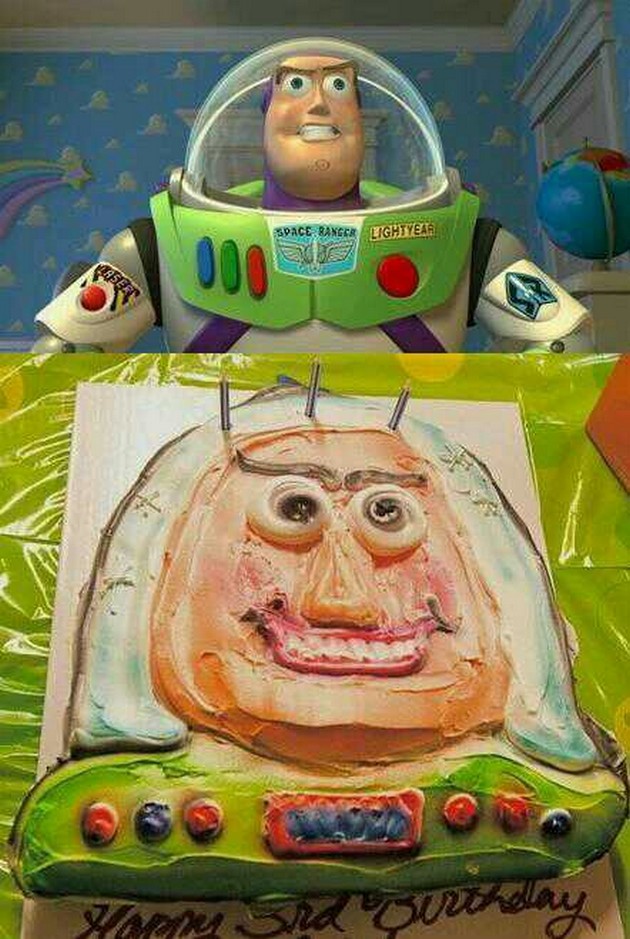The image showcases a humorous baking fail, depicted in a two-part composition. At the top is a still from the movie Toy Story, featuring Buzz Lightyear wearing his iconic green and white space suit, standing with his arms outstretched, staring off into the distance. His surroundings hint at a child's room, with blue wallpaper adorned with clouds and a globe positioned to his right. Below this screenshot is a photograph of a birthday cake attempting to replicate Buzz Lightyear's likeness. Instead of capturing Buzz's heroic demeanor, the cake presents a distorted, terrifying version of his face with disproportionately large, bulging eyes and a demonic-looking smile. The cake is primarily green to mimic Buzz's armor, with his peach-colored face appearing poorly crafted and smudgy. Three candles are placed on top, where Buzz’s helmet would be, and at the bottom of the photograph is a message that reads "Happy Third Birthday," referencing the occasion. The cake rests on a green table mat, further tying it to Buzz's color scheme. Overall, the contrast between the confident, animated Buzz and the unsettling cake provides a comically stark comparison.